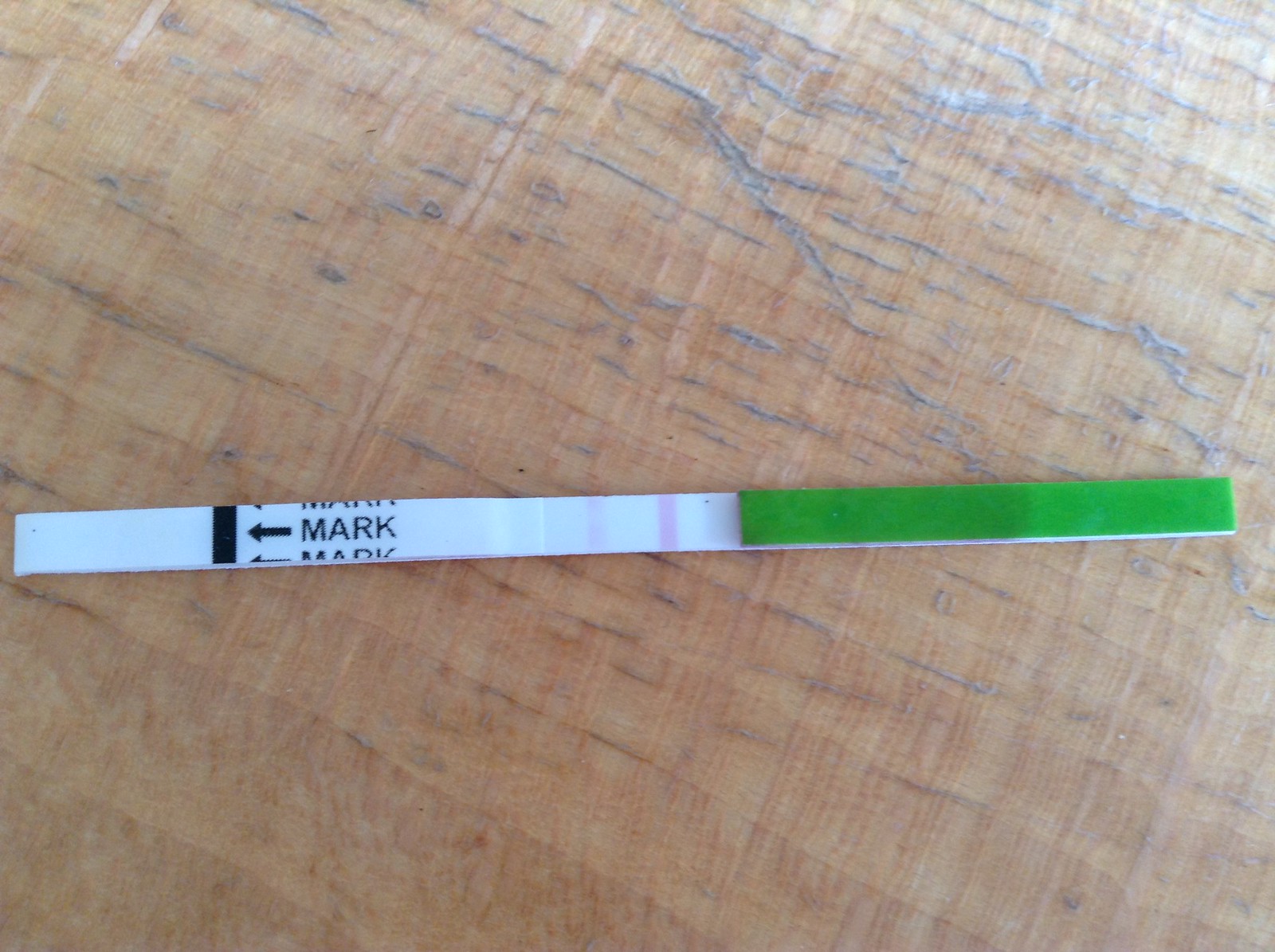The image depicts a long, stick-like object that could be a marker or a dipstick used for measurement purposes. The stick has a white base and a green-colored end, with the green section covering approximately one-third of its length. There are pink lines or marks spaced across the white portion of the stick, suggesting it serves a specific measurement function. The word "MARK" is clearly printed on the white part of the stick, and arrows point toward a thick black mark across it. The green section varies in shade, being darker in some areas. The stick is placed on a table with a visible wood grain texture and distinct markings. Although the specific use or substance being measured by the stick is not indicated, the presence of these markings suggests a precise and intentional design.